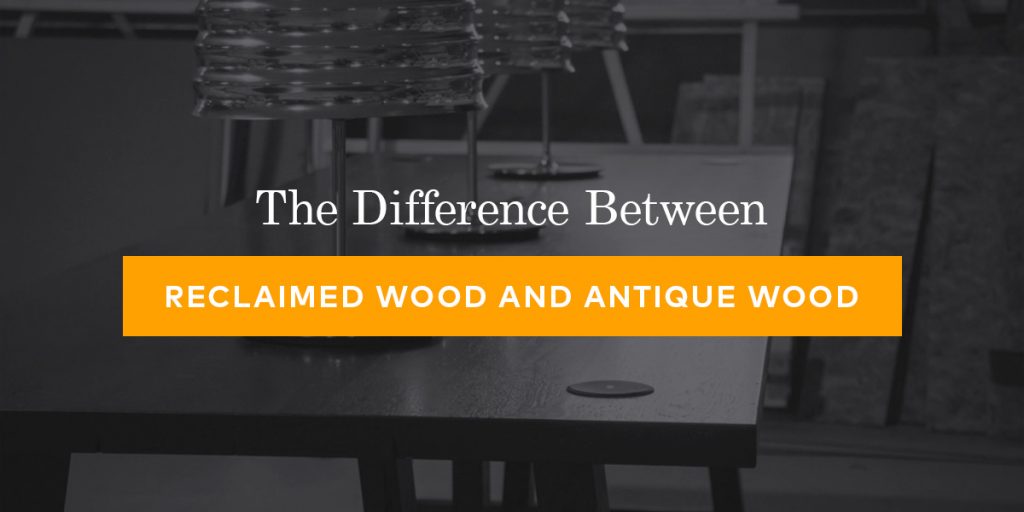The image is a darkly filtered, almost black-and-white photograph, primarily featuring a wooden tabletop in the foreground and wooden boards in the background. Centered both vertically and horizontally on the image is white text that reads, "The difference between." Below this phrase, there's an orange stripe with white, uppercase lettering, "RECLAIMED WOOD AND ANTIQUE WOOD." The setting appears to be a desk, possibly part of a website display aimed at contrasting reclaimed wood (which implies recycled material) with antique wood. Despite the dark tones of the photograph, the text is clearly readable, emphasizing the distinction between the two types of wood through the centered and highlighted design elements.